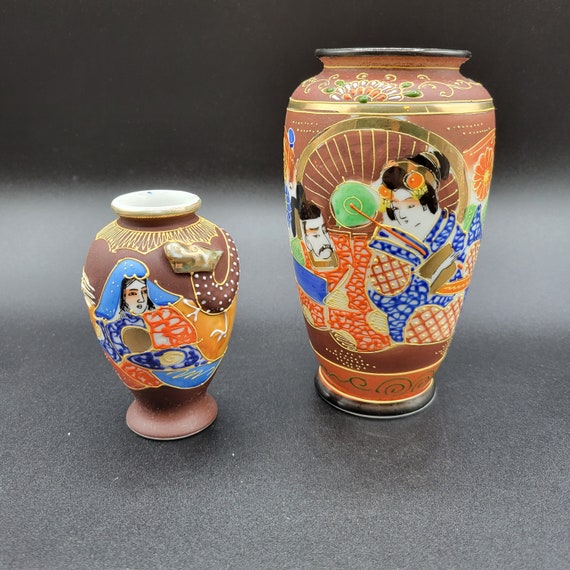The image showcases two intricately designed, antique oriental vases placed on a grayish surface that fades out of focus towards a black background. The taller vase on the right, which occupies about two-thirds of the photograph, features elaborate decorations including shiny gold insets and artwork depicting a man and a woman dressed in traditional kimonos and Japanese headgear, either conversing or eating, with a prominent orange border at the bottom. The shorter vase on the left, capped with a top, displays a detailed painting of an oriental woman adorned in blue and red robes and a blue headdress, gazing at a brown dragon. Both vases, primarily brown in color, are adorned with various colors including blue, orange, and gold, adding to their ornate and antique appearance.